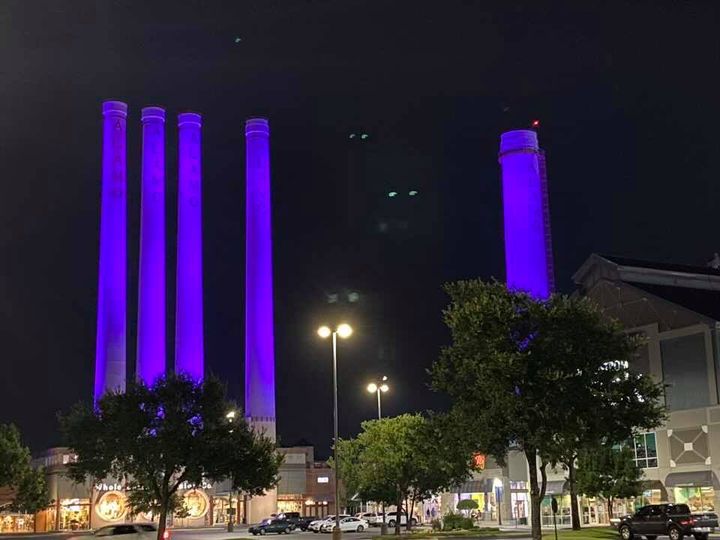The photograph showcases a nighttime scene at a shopping center, with a parking lot featuring several cars, predominantly white and black, illuminated by street lamps. The foreground is adorned with about five to six trees, partially concealing the storefronts, though a Whole Foods might be among them. The sky is pitch-black, adding to the contrast of the well-lit area. In the background, five tall factory chimneys, brightly lit in purple, tower above the scene, reaching almost to the top of the image and dwarfing the surrounding buildings. Despite the late hour suggested by the dark sky, the vivid lighting of the buildings and the presence of people on the sidewalk indicate that the shopping center is still active.